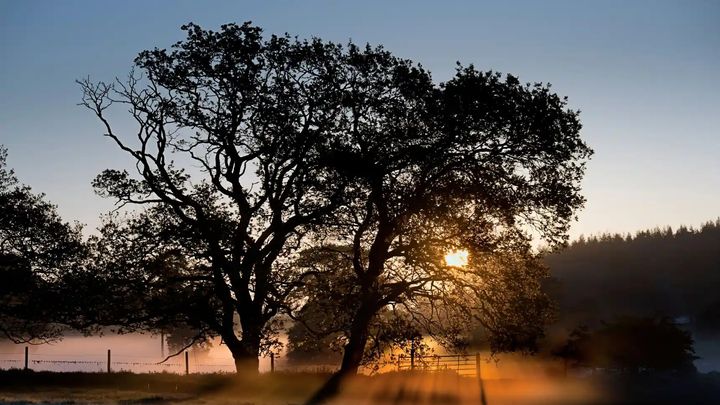The image captures a picturesque sunset scene featuring a large, silhouetted tree as the focal point. The sun, setting in the background, casts a beautiful orange and yellow glow across the sky, filtering its light through the darkened branches and leaves of the tree, rendering them almost black due to the shadows. This dramatic interplay of light creates beams through the foliage, adding a striking contrast. The tree stands amidst scattered evergreens and mature trees, all bathed in the same warm hues of the setting sun. Below the tree, a fence—likely an electric one—suggests the presence of livestock, even though none are visible. At the base of the image, a faint mist or fog is noticeable, adding a layer of ethereal beauty. The overall scene is framed by patches of darkened trees on the sides, with the vibrant orange sun peeking through the branches as it dips lower, almost touching the horizon.